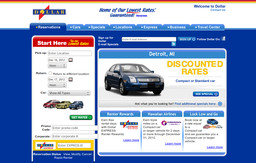A screenshot of an outdated automobile website is displayed, characterized by its predominantly blue background. The site appears to specialize in car sales, possibly focusing on vehicles offered at discounted rates. At the top of the page, the title simply reads "Dollar" against a white backdrop. Below the title, a search bar is prominently featured, accompanied by a navigation panel on the left, which likely allows users to search for cars by make, model, and year. 

The center of the page showcases a few cars, presumably sedans, one of which is blue and highlighted with the text "discounted rates" on a white background. Three additional sedans are displayed in a row, colored red, yellow, and blue. The top of the site features a white banner with various links, though the text is too small to be readable. Given the emphasis on discounted rates, it is inferred that the site might be focused on selling used cars.